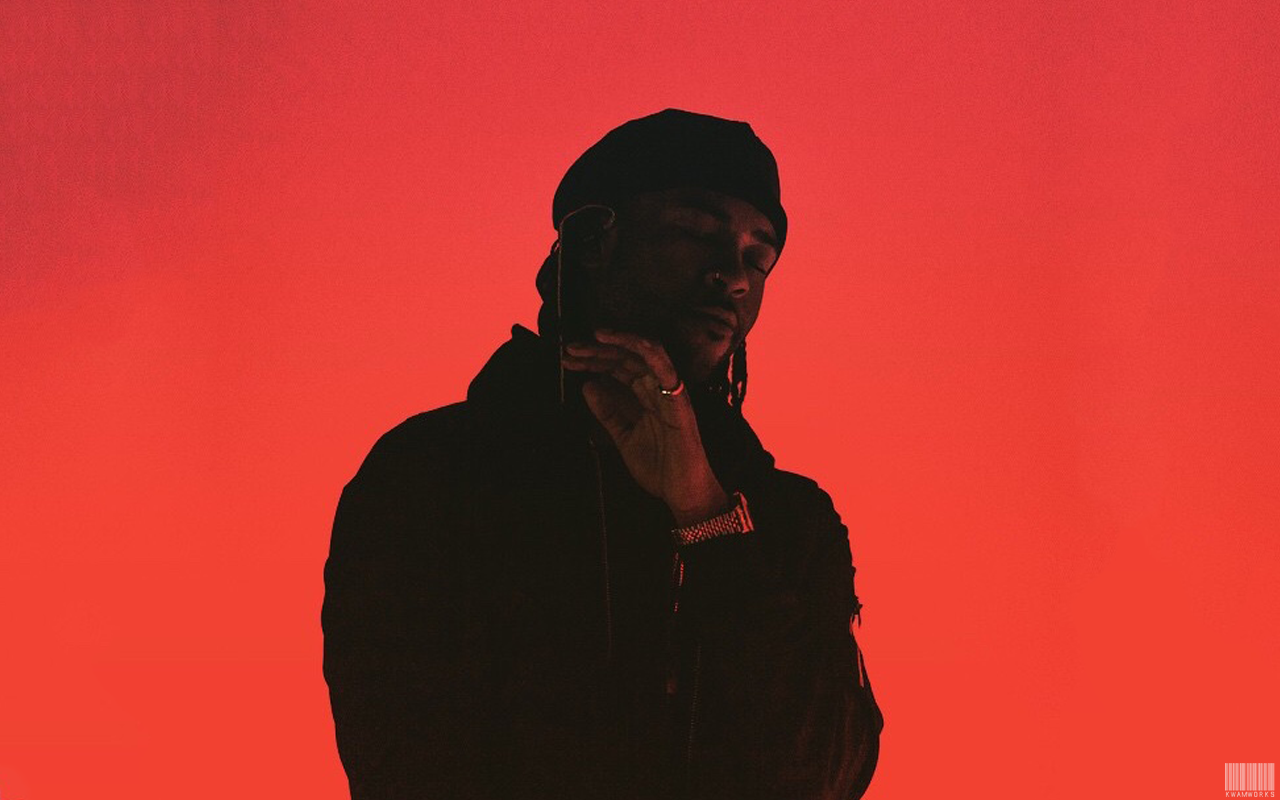The image appears to be an album cover featuring a black man, possibly a musician. The striking background is a vivid red, creating a dramatic contrast with the darker, shadowy figure at the center. He is illuminated from below, highlighting his features against the intense backdrop. The man, who has long dreadlocks, wears a dark hat and a combination of a hoodie and a long-sleeve black jacket. His eyes are closed, his head slightly tilted downward. His left arm is bent at the elbow, with his hand raised in front of his face, displaying a pinky ring and a gold watch. He also has a nose ring in his right nostril. In the bottom right corner, there is small white text and a barcode, possibly identifying it as an album cover. The text includes the initials "KW A.M. Works."